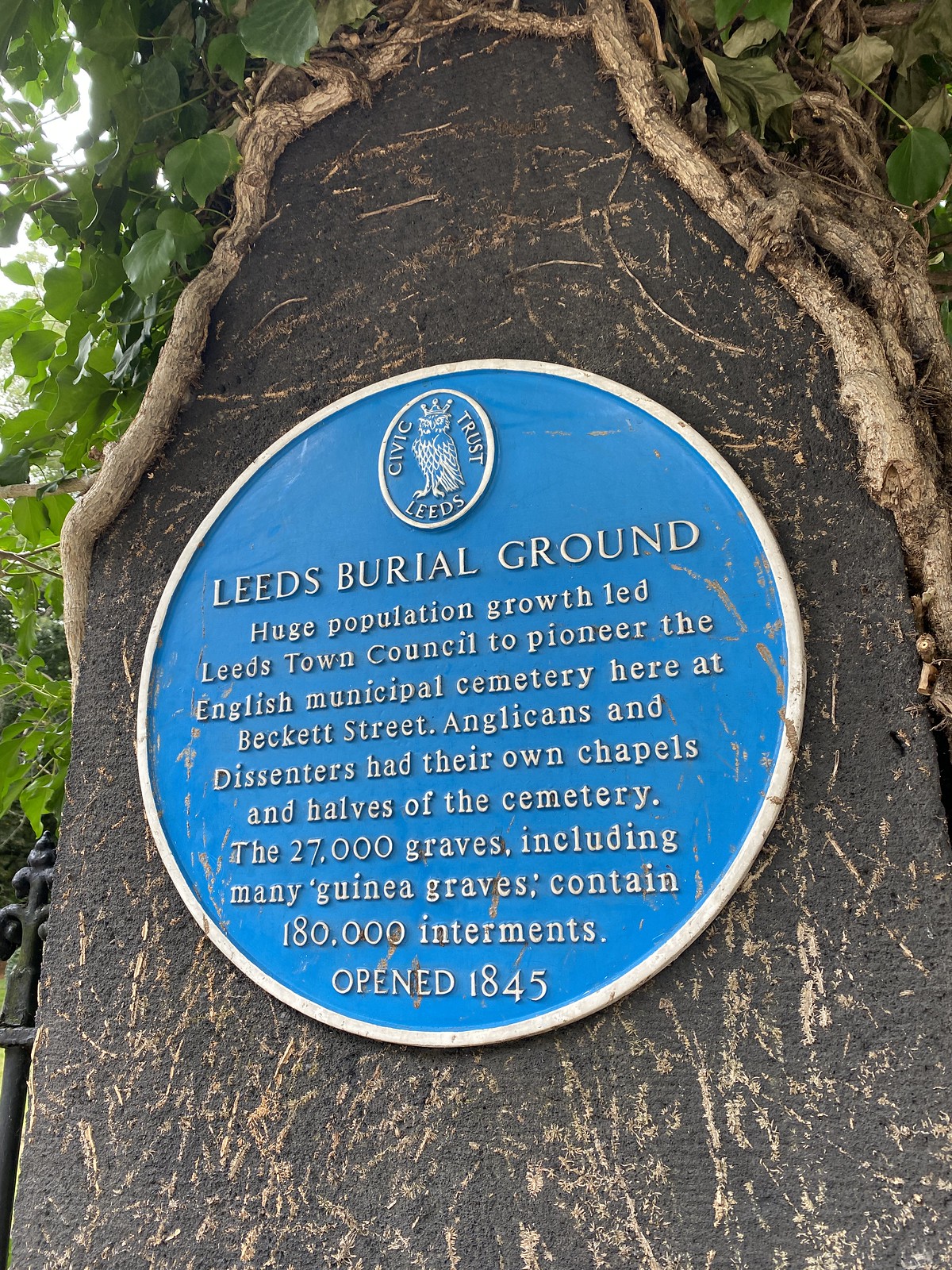This is a vertical photograph of a historical blue plaque mounted on a stone plinth, overgrown with vines and leaves. The stone plinth appears weathered, reflecting its age and the historical significance it denotes. The blue plaque is circular, featuring a white border, white lettering, and the white crest of the Civic Trust Leeds, which includes an owl in the center. The inscription on the plaque reads: "Leeds Burial Ground. Huge population growth led Leeds Town Council to pioneer the English Municipal Cemetery here at Beckett Street. Anglicans and dissenters had their own chapels and halves of the cemetery. The 27,000 graves, including many Guinea graves, contained 180,000 interments, opened 1845." This photograph was captured during the day under overcast skies, ensuring natural but diffused lighting without direct sunlight. The alignment of the image is portrait.